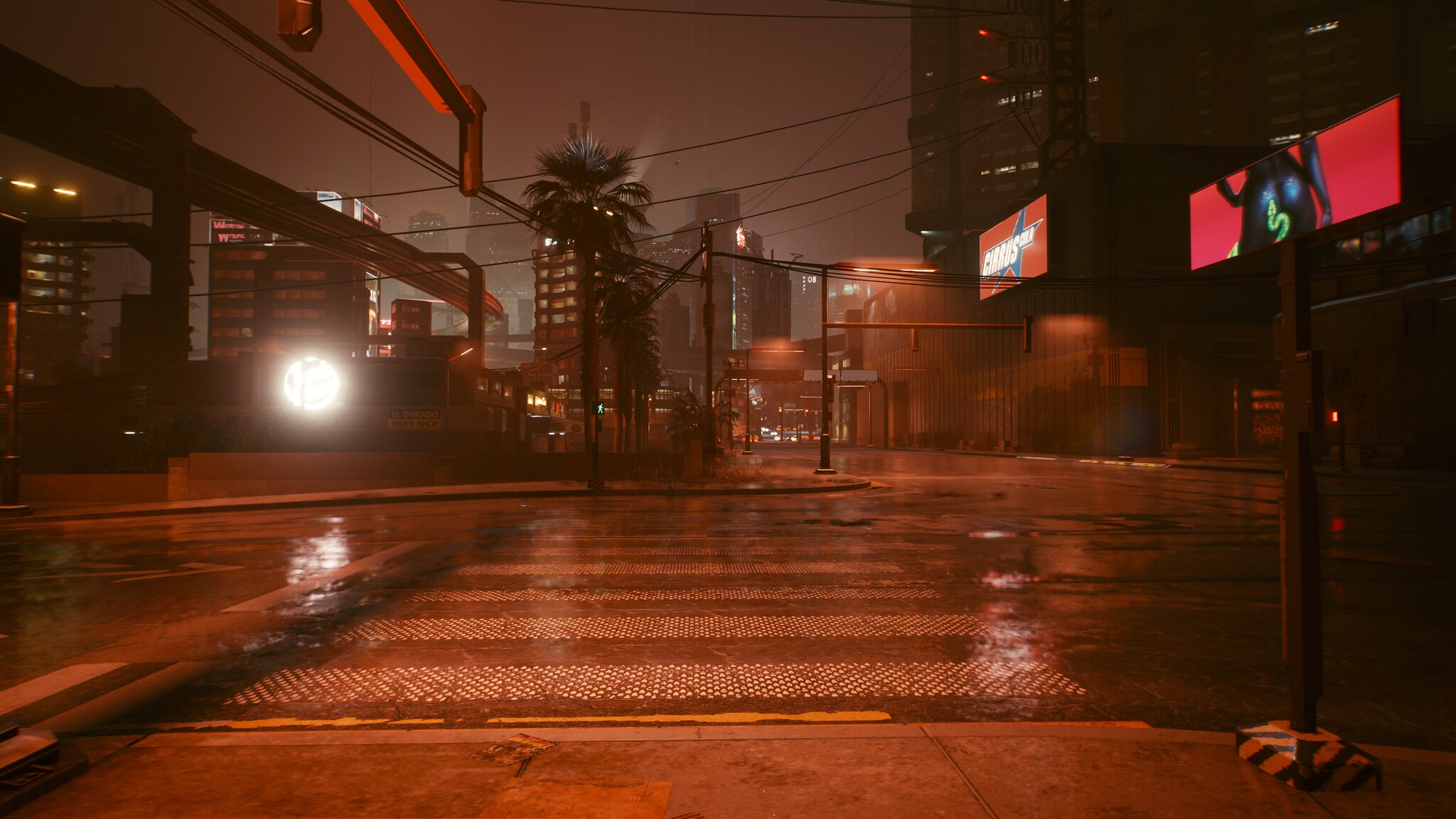This nighttime photograph captures a rainy city intersection in a downtown area illuminated by various lights. The wet pavement reflects these lights, enhancing the moody ambience of the scene. Prominent in the foreground is a white-striped pedestrian crosswalk leading into the intersection, emphasizing a moment of stillness. Large buildings, silhouetted against the night sky, rise in the distance, framing the scene with a sense of depth and urban scale.

To the left, a high and bright light suggests the presence of an elevated structure, possibly train tracks or a monorail, adding an element of industrial activity. Multiple illuminated billboards and LED screens display advertisements, adding vibrant, albeit unreadable, splashes of red, green, blue, and white to the landscape.

A solitary palm tree, its silhouette stretching above utility wires, stands near the crosswalk, a contrast to the urban environment and a reminder of nature's adaptability. Overhead lighting casts reflections on the street, further highlighting the wet conditions. The intersection and empty street impart a feeling of solitude amidst the urban expanse, punctuated by the distant skyscrapers and the quiet after the rain.